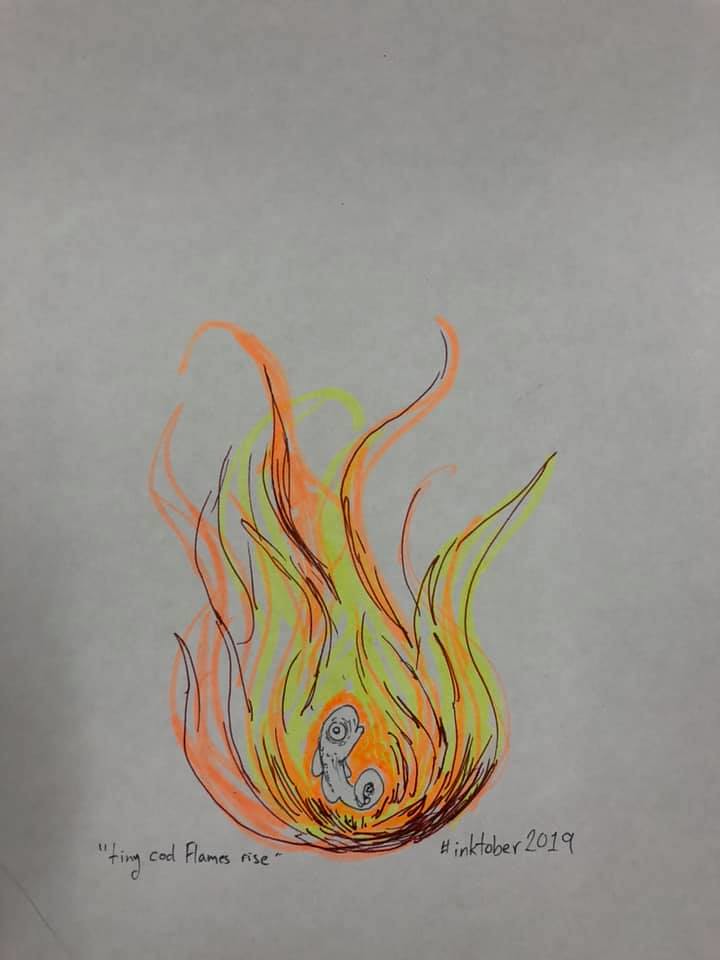This image features a detailed, hand-drawn illustration on a white or light gray piece of sketch paper. The drawing, centered towards the bottom of the page, depicts a large flame with a dark pen outline, filled with vibrant swirls of orange and yellow to simulate fire. Nested within the flame is a small, distinct creature resembling a codfish or tadpole. The fish is characterized by its large circular eye, upward-facing head, curved body, and slightly curled tail. Notably, handwritten inscriptions accompany the drawing: on the left side at the bottom, in quotations, it reads "Tiny Cod Flames Rise," with only the 'F' in "Flames" capitalized; on the right side, it states "#InkOctober 2019" in small letters. There is also a subtle shadowing effect on the paper's left side, enhancing the overall depth of the drawing.